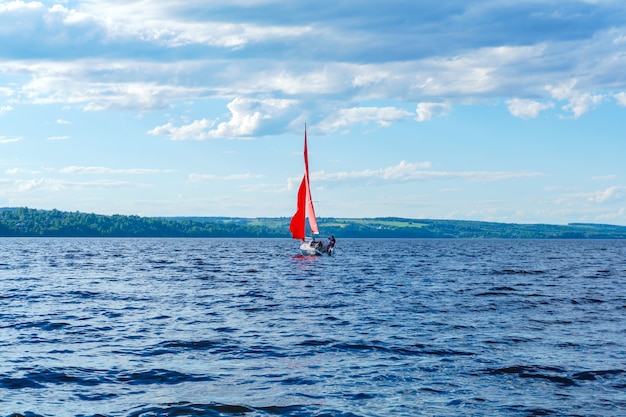The image features a large, serene body of water, possibly a lake or river, where small, gentle waves ripple across the rich blue surface under a daytime sky. Though clouds are present, sunlight filters through, lending a soft light to the scene. Situated in the middle of the water is a white sailboat with two distinct red sails, appearing to tilt as if affected by a disturbance. A person, possibly guiding the boat, is noticeable at its front, and there seems to be a suggestion of movement indicating someone might be falling into or entering the water. The background reveals a lush, green landscape dotted with forests and small hills, adding to the tranquil yet dynamic atmosphere of the image.